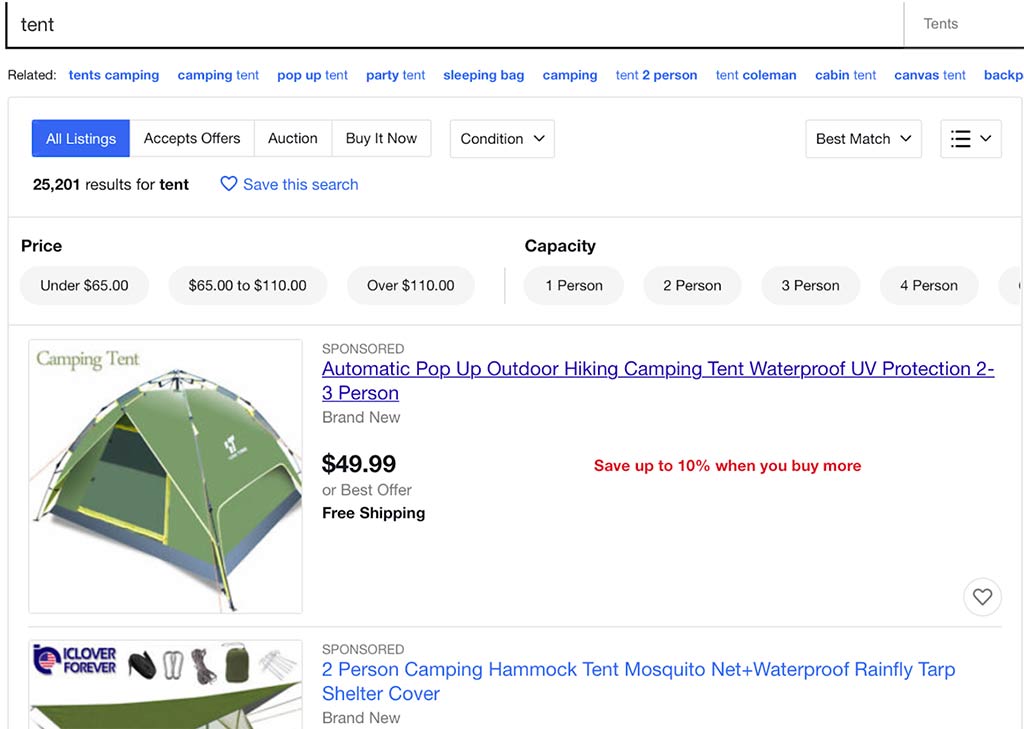This is a detailed screenshot of an eBay search page. Visible at the top left corner is the familiar eBay logo, with the search bar prominently displaying the user's query: "tent." The user is searching under the category "tents," as indicated in the top right corner.

Under the search bar, eBay has provided related searches such as "tents camping," "camping tent," "pop-up tent," "party tent," "sleeping bag," "camping," "tent two-person," "tent Coleman," "cabin tent," "canvas tent," and "backpacking." Further down, several buttons allow users to filter their view: "All Listings" is highlighted in blue, with additional options for "Accept Offers," "Auction," and "Buy It Now." Users can also adjust the condition and sort results by "Best Match," both accessible via drop-down menus, and use a "sandwich" icon to access more settings.

An impressive total of 25,201 results appear for the search term "tent." A blue button labeled "Save this search" with a heart icon allows users to save the search. Price filters include options for "Under $65," "$65 to $110," and "Over $110," alongside capacity filters ranging from "1 to 4 Person" and possibly more.

The first two posts listed are sponsored. The first sponsored post features a green tent in an image on the left. The listing is for an "Automatic Pop-Up Outdoor Hiking Camping Tent," offering waterproof and UV protection for 2 to 3 persons. It is listed as brand new, priced at $49 or best offer with free shipping, along with a note about a 10% discount for multiple purchases.

The second sponsored item is a green two-person camping hammock with a mosquito net, plus a waterproof rain fly tarp shelter cover, also described as brand new. Only a partial image of the hammock is visible. These are the key details captured in the screenshot.